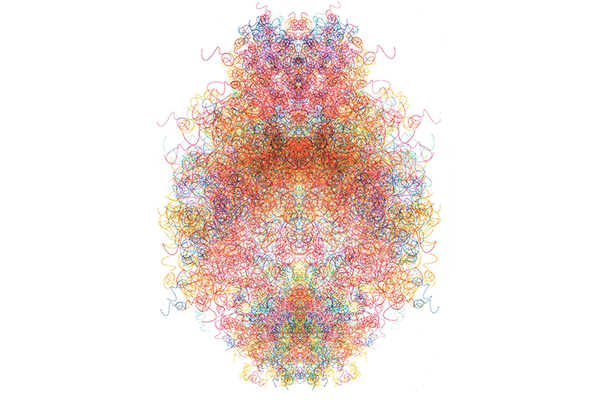The image is a close-up of an abstract, colorful line drawing characterized by intricate interwoven strings of varying densities. The lines, resembling curlicues or spirals, include an array of hues like red, blue, yellow, orange, green, cyan, purple, and pink, creating a vibrant tapestry. The composition forms a tall, oval to diamond shape with a white background partially visible through the less dense areas.

Central to the image is a dense concentration of red, pink, cyan, and blue lines, giving it a rich, textured look. At the top, the lines are primarily cyan with interspersed green, while the bottom showcases a mix of cyan and green bordered by red squiggly outlines. The entangled lines and squiggles meander in all directions.

The overall pattern could be interpreted as an artistic representation of a brain or a face, hinted by the density and arrangement of the lines which create shapes reminiscent of a downward-facing skull. This has heavier shading towards the center and the top, which tapers off to more delicate, spaghetti-like strings along the edges. The visual density varies, providing a central focal point with a delicate, airy perimeter.